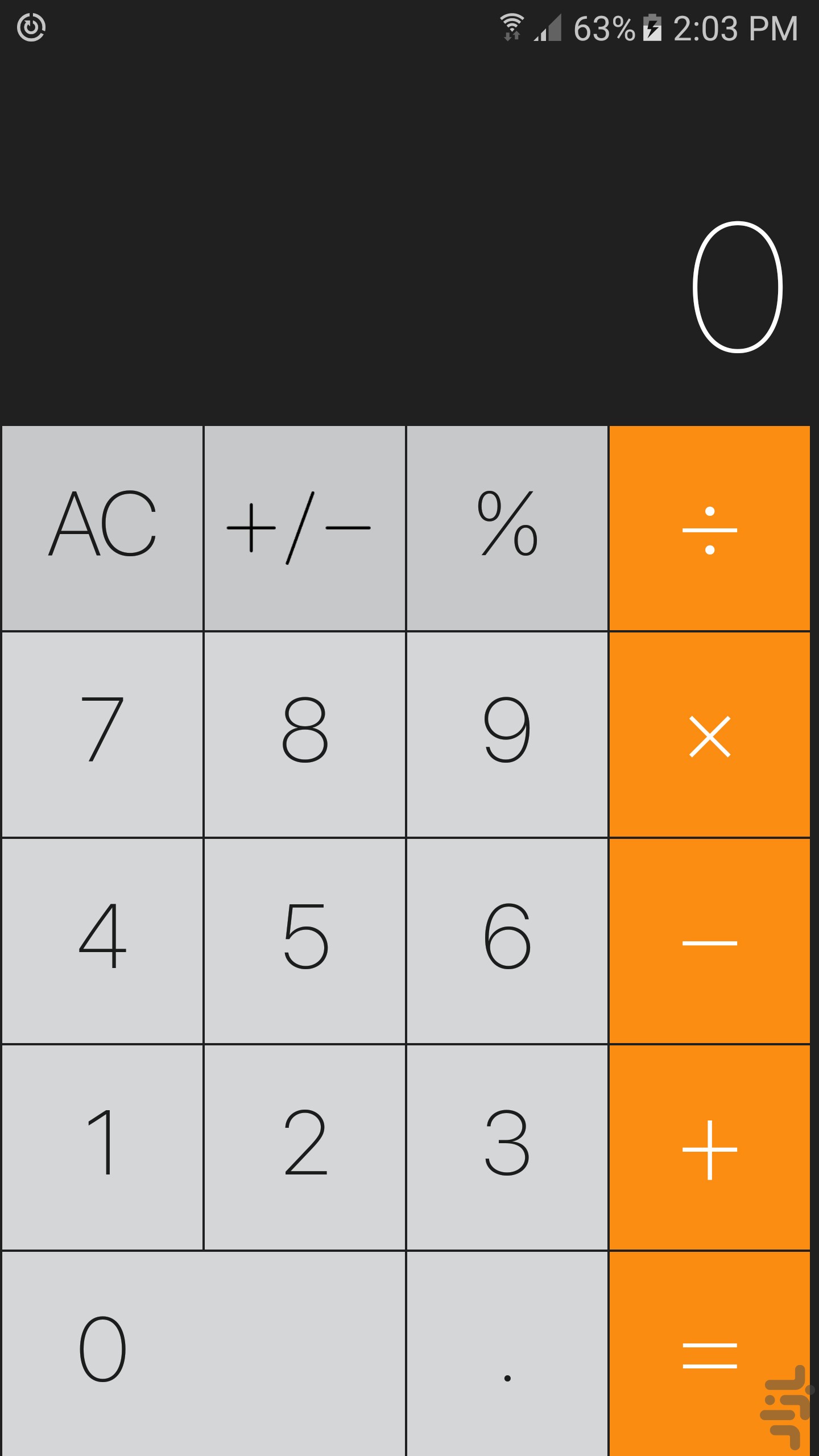The image is a screenshot of a smartphone calculator app displayed on a device with 63% battery and full Wi-Fi hotspot signal at 2:03 PM. The background of the calculator interface is black, with most numeric and functional keys in white lettering. The zero is currently displayed on the screen. 

On the right side of the interface, the function keys for division, multiplication, subtraction, addition, and the equals sign are all set in orange boxes with white text. The left and middle sections feature keys in gray boxes with white labeling, arranged as follows from top to bottom: 

- Top row: "AC" (all clear)
- Second row: "7", "8", "9" 
- Third row: "4", "5", "6" 
- Fourth row: "1", "2", "3" 
- Fifth row: "+/-" (for toggling positive/negative), "0", and a period (.) for the decimal point

This specific calculator app appears to be a standard one, likely the default application included with many Android devices. The app has a straightforward design, providing all basic arithmetic functions.